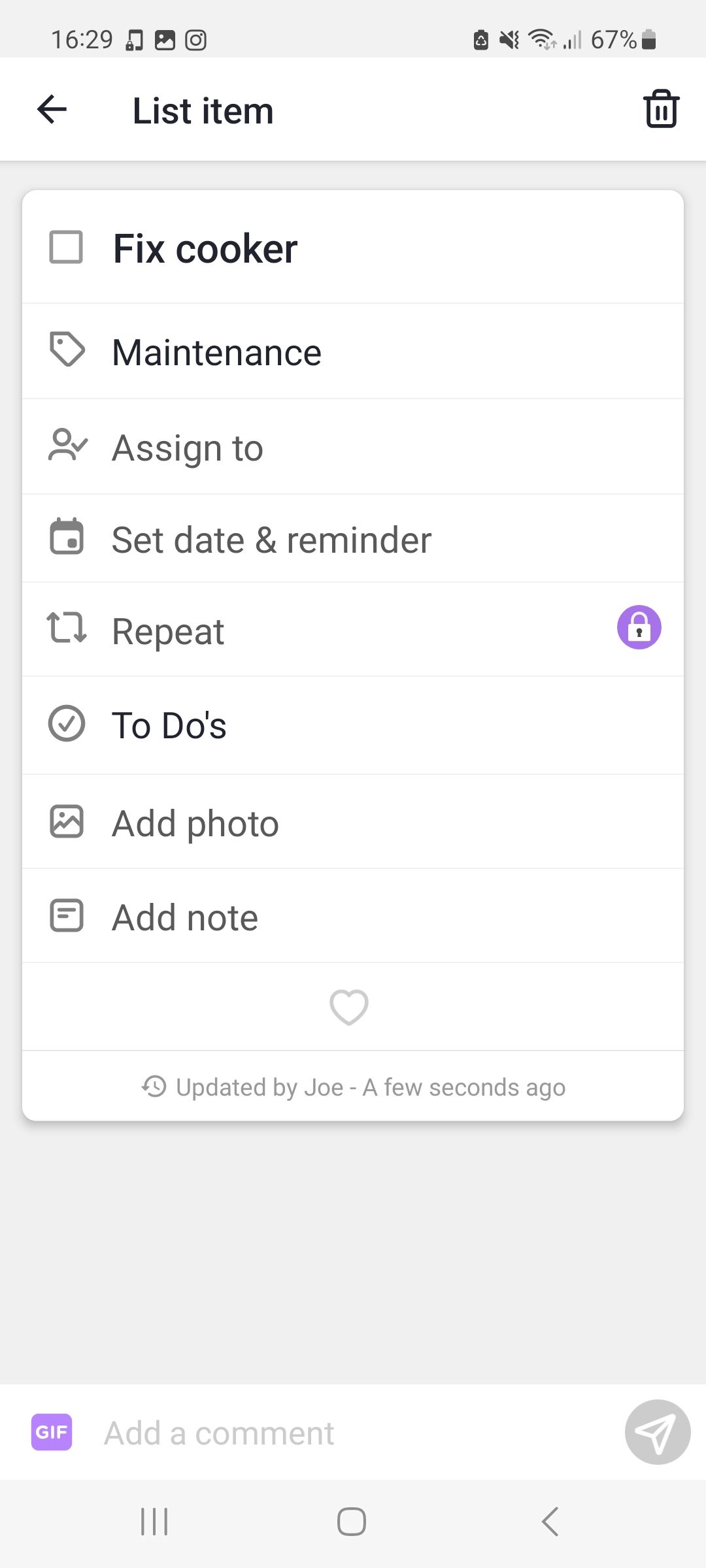In this detailed screenshot of a cell phone interface:

- The background features a clean white and light gray color scheme.
- The upper left corner of the screen displays the current time as 16:29.
- The upper right corner shows a battery icon with 67% charge remaining and a Wi-Fi connection with two out of four bars.
- Below the status bar, there is a list item featuring a leftward-pointing arrow and a trash can icon to the right, indicating options for navigation and deletion.
- Subsequently, a white box contains text reading "Fix Cooker," accompanied by a small square image on its left side.
- The section is labeled "Maintenance," indicating the task category.
- Below that, there is the "Assign To" option, iconified by a person silhouette with a checkmark, suggesting task delegation.
- The "Set Date and Reminder" feature is represented with a calendar icon on its left.
- The "Repeat" function is denoted by upward and downward pointing arrows.
- Towards the right, in a highlighted purple circle, there is a white lock icon, possibly indicating task security or privacy settings.
- Further down, a “To Do’s” section features a gray checkmark within a circle.
- At the bottom, there are options for "Add Photo" and "Add Note" for additional task details.

The overall layout is methodically organized with intuitive icons, making task management straightforward.